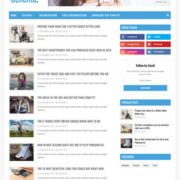A very blurry screenshot of a webpage, making it impossible to discern specific details or read any text. The layout features a sky blue section in the top left corner with unreadable text. In the center top, only the bottom edge of an image is visible. The upper right corner contains something gray, beneath which spans a sky blue banner with five indistinct white labels. Running down the right side of the page are various bars, seemingly dividing the content into categories. Among these are two columns, each with three rows of colored icons—purple, orange, and pink on the left, and blue, orange, and gray on the right. Below these is some text above a blue line with white writing, continuing down the page. The main content area on a white background consists of eight rows of images, each accompanied by a paragraph of black text, both heavily blurred.